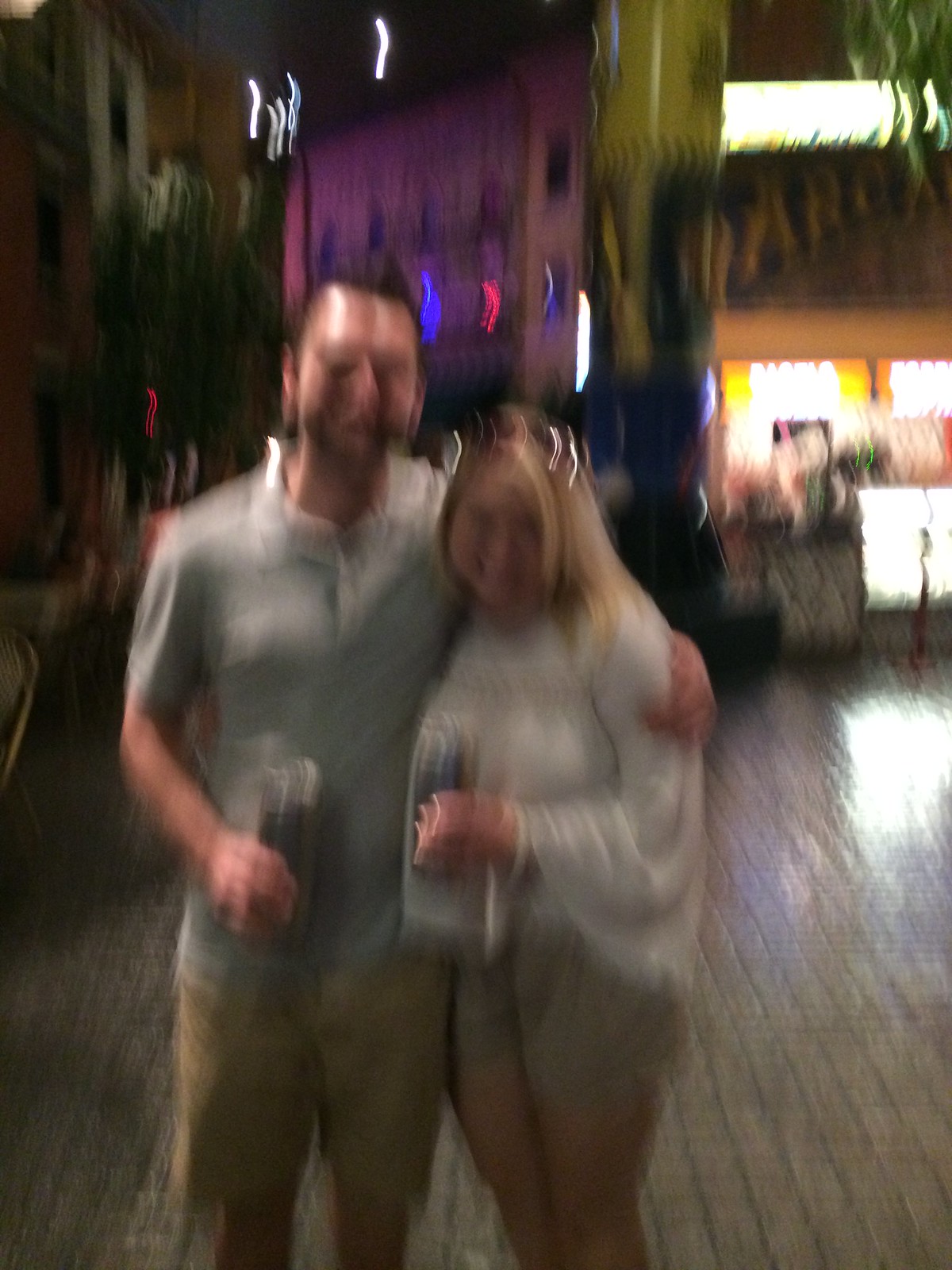Blurry nighttime photograph capturing a joyful moment between an attractive Caucasian couple, both holding alcoholic drinks. They are embracing each other, surrounded by a lively backdrop of shops and bars, all indistinct due to the blur. The man, sporting a blue polo shirt and khaki shorts, has brown hair with a widow's peak. The woman, dressed in khaki shorts and a white top, has blonde hair. They are standing on a tiled floor, clearly enjoying their outing together.